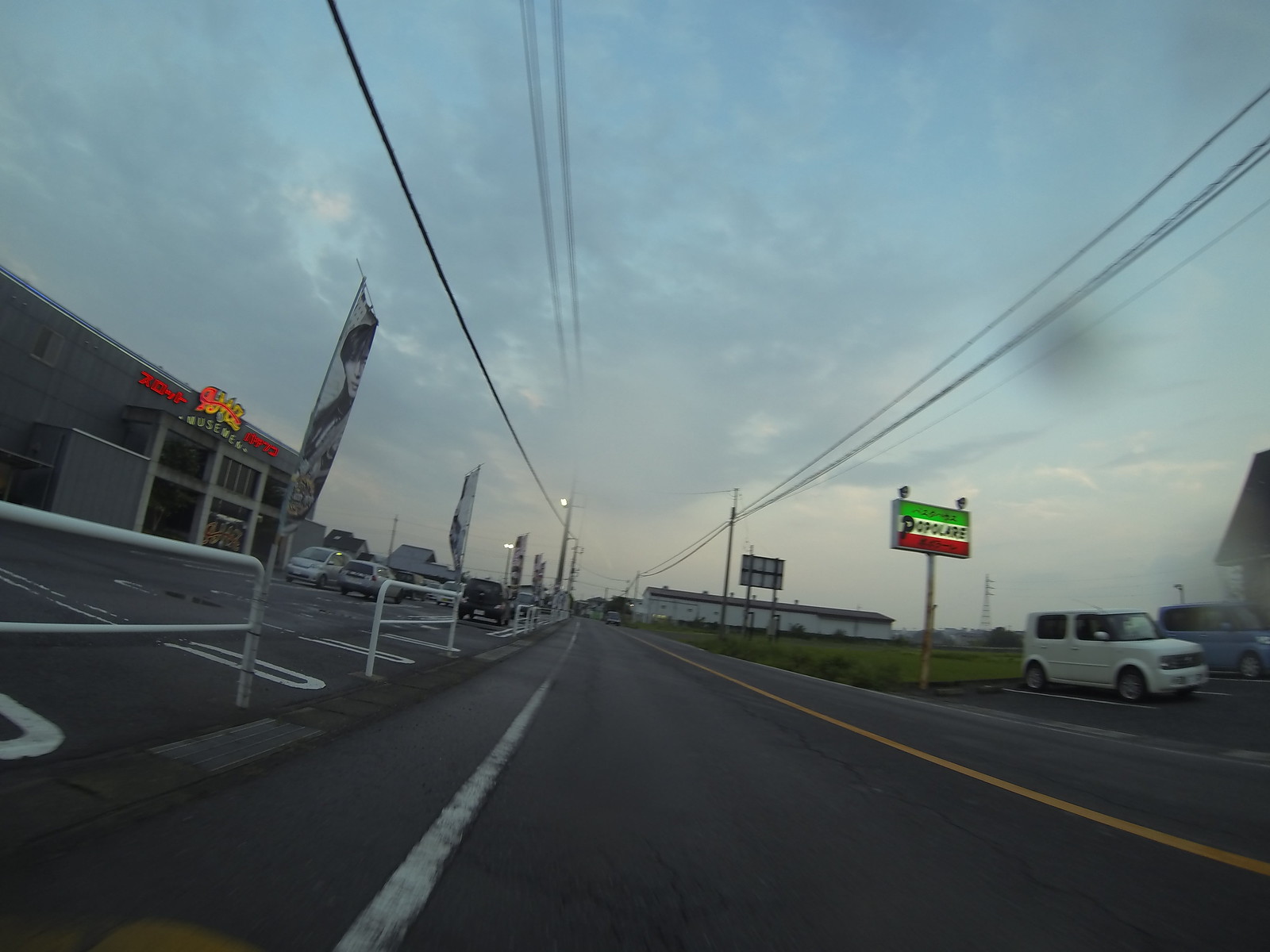This image captures a bustling street scene at dusk, with the sky transitioning to night beneath a canopy of clouds. On the left side of the road stands a prominent building, which appears to be a museum. The facade displays either Chinese or Japanese characters, hinting at the cultural significance of the institution. Vehicles are parked along both sides of what seems to be a one-way street. Illuminated under the dimming sky, a sign with the word "Popular" hangs on the right side of the image, adorned with a tricolored flag featuring green, white, and red vertical stripes, reminiscent of either the Italian or Mexican flag. A white vehicle and a blue vehicle are parked in front of what looks like a restaurant near the sign, adding a sense of liveliness to the scene.